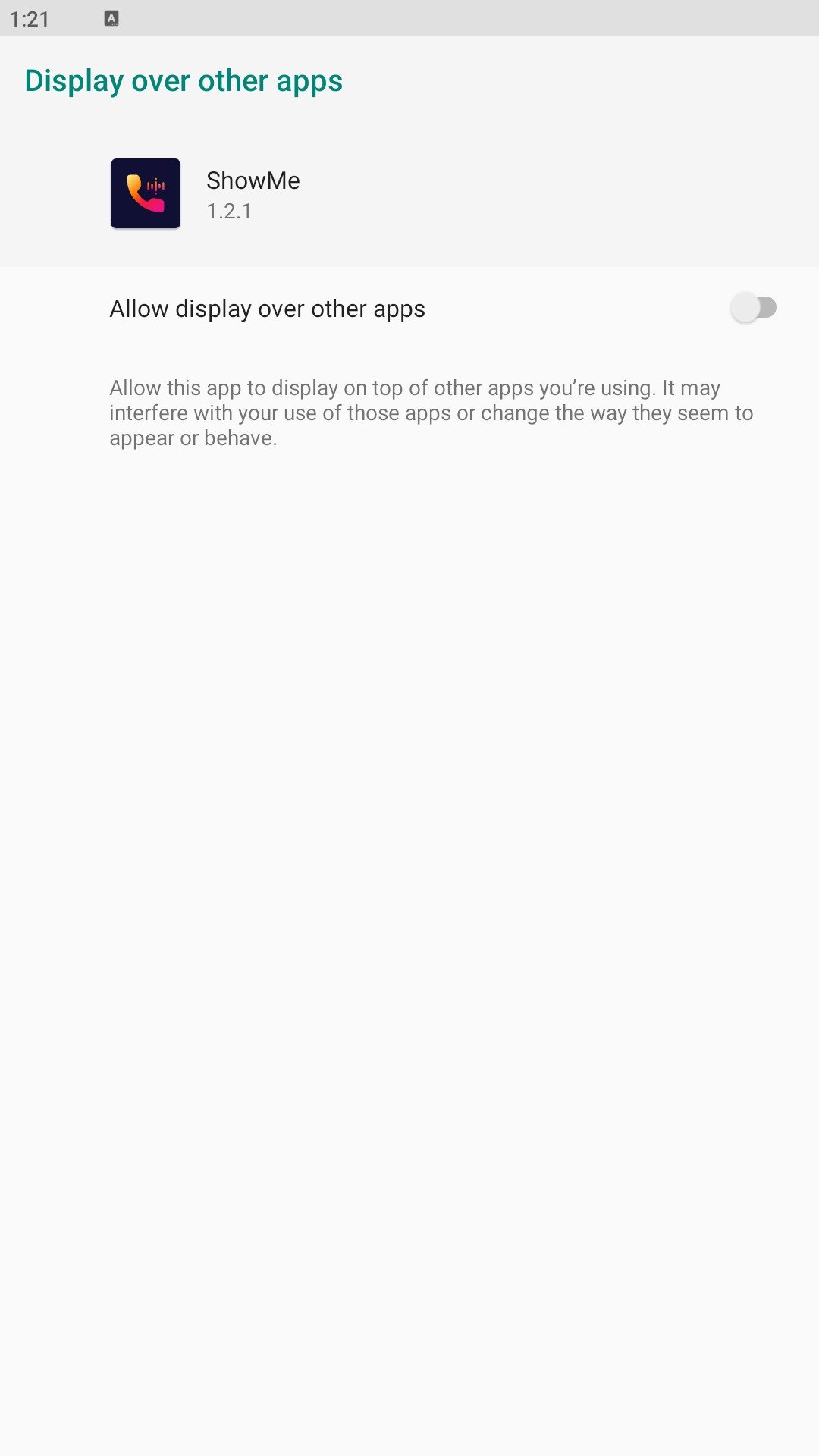This screenshot features a user interface configuration screen. In the upper left-hand corner, the time reads "1:21". Directly beneath this, on the left side, there is a section titled "Display over other apps". Below this title, there is a phone icon symbol. To the right of this symbol, the text "Show me 1.2.1" is displayed. 

Further down, there is a toggle option labeled "Allow display over other apps" with an on/off switch positioned on the right side, currently set to "off". Below this toggle option is a detailed explanation: "Allow this app to display on top of other apps you're using. It may interfere with your use of those apps or change the way they seem to appear or behave."

The background behind this informative section is a light gray color, which contrasts with the darker gray color used for the paragraph text. The "Allow display over other apps" text is rendered in a darker black font, emphasizing its importance, while the toggle button retains a gray color, indicating it is currently in the "off" position. The remainder of the screen is blank, dominated by the light gray color.